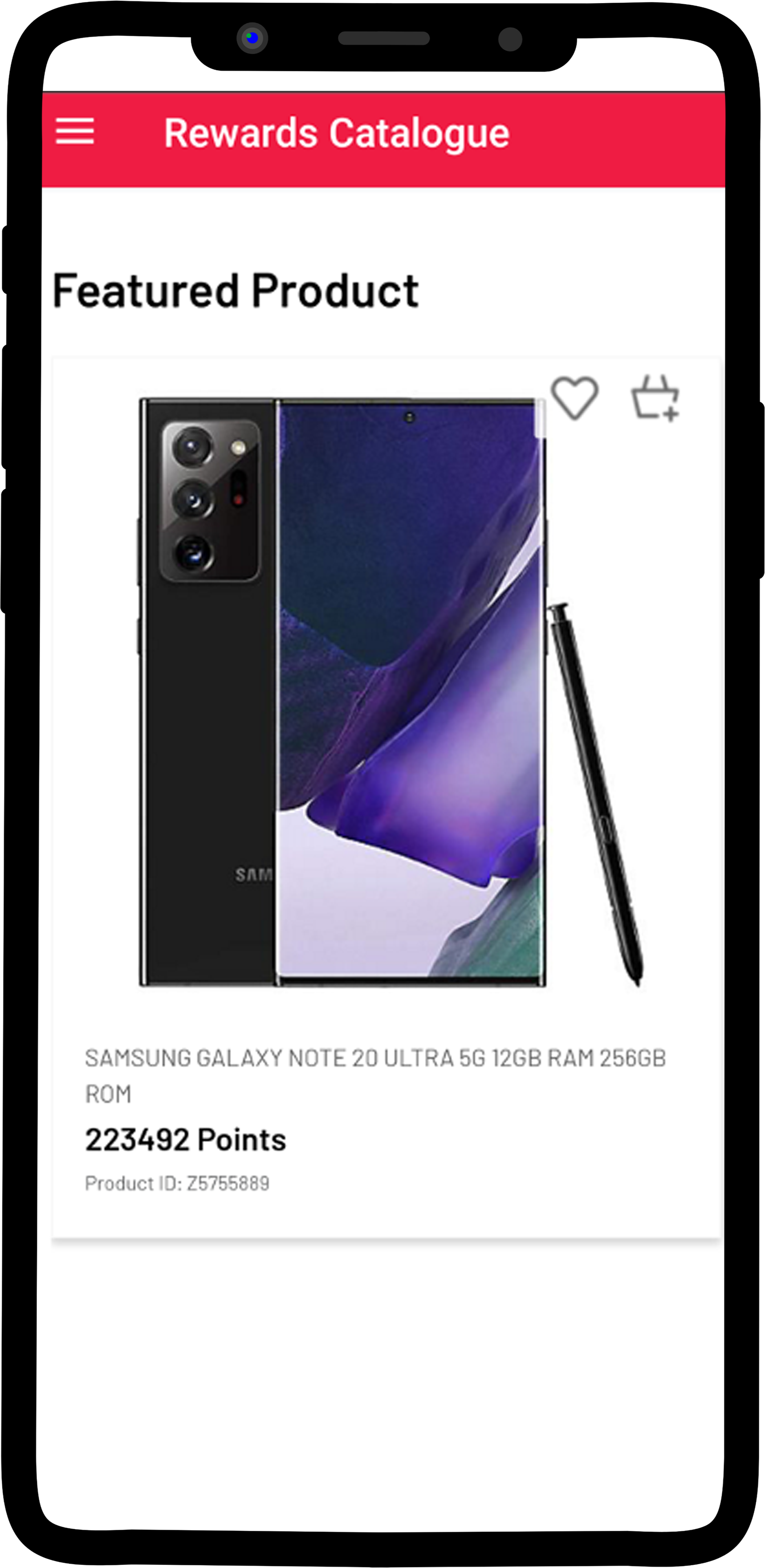The image showcases a black cell phone prominently placed against a white background. The phone features visible side buttons and a distinct red strip at the top of its display. The screen shows an interface with the words "Rewards Catalog" in white, beneath which "Featured Product" is written on a white background.

The display details the item being featured—a Samsung Galaxy Note20 Ultra 5G. The image provides a view of both the front and back of the device, with a stylus propped up against the right side. In the upper right corner of the screen, there's an icon of a heart and a shopping bag with a plus sign on a white background.

Below the product image, text in gray reads: "Samsung Galaxy Note20 Ultra 5G, 12GB RAM, 256GB ROM," followed by "22, 33, 34, 92 points" and the "Product ID: Z5755889." A gray line is present beneath this information. The phone's display features a colorful screensaver with shades of blue, light purple, dark purple, navy blue, and green. The back of the phone is solid black.